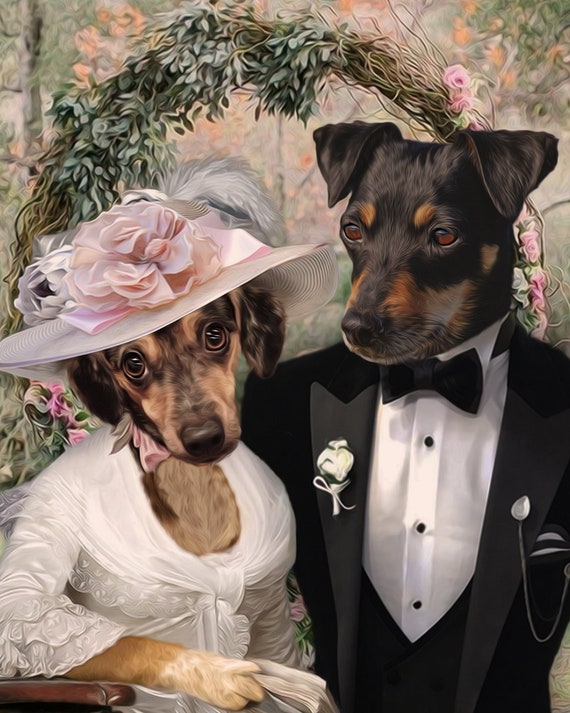The image is a painting of a wedding scene featuring two dogs standing as a bride and groom in front of a blurred background with an archway made of green foliage and pink flowers. The dog on the left, acting as the bride, is a light and dark brown dog with slightly longer folded ears. She is elegantly dressed in a silky white wedding dress with lace details and is wearing a large pink hat adorned with flowers, tied under her chin with a ribbon. In her paw, she appears to be holding a fan, and she leans against a brown counter. The groom dog, positioned on the right, is black and brown with folded ears and is wearing a black tuxedo with small buttons and a black bowtie, complemented by a white boutonniere. Together, they form a whimsical and detailed portrayal of a canine wedding.